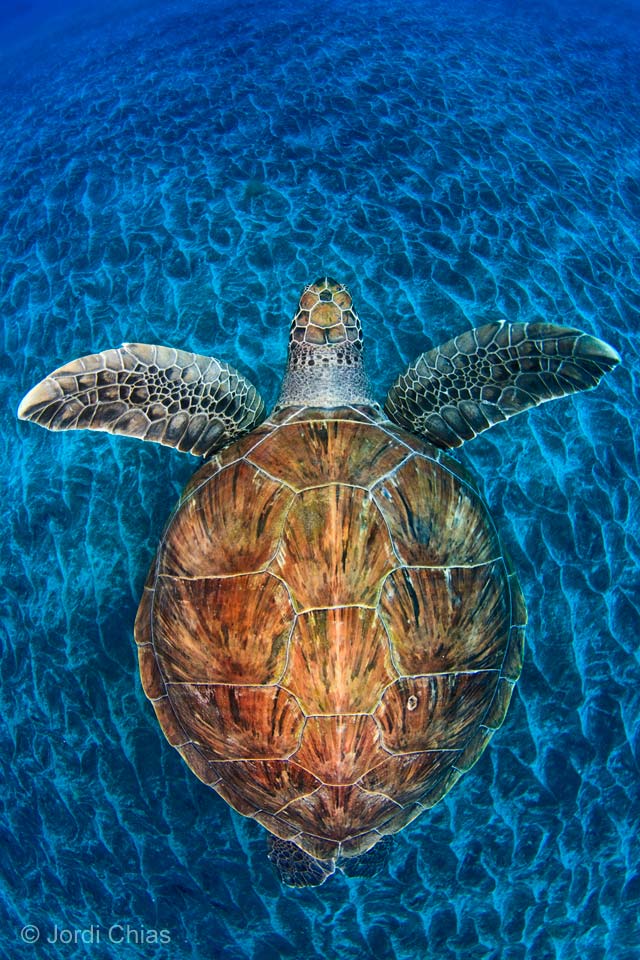This is an ultra high-definition image featuring a large sea turtle swimming in crystal-clear, aqua blue waters. Captured from a top-down perspective, the turtle's detailed and intricate shell markings, resembling black and brown pebbles, are clearly visible, as are the textured patterns on its head and flippers. Its flippers are extended in a T-shape, displaying an olive green, almost brownish hue. The turtle's face and short neck have a brown and gray coloration respectively. The clarity of the water below creates ripples, giving an impressionistic effect that almost resembles a painting. This image might be a photograph or a very detailed artwork, but its quality is undeniably superior. In the bottom right corner, there is a copyright watermark that identifies the creator as Jordi Chias. The water appears both light and dark blue, indicating a shallow area that is immaculately clean and well-maintained.